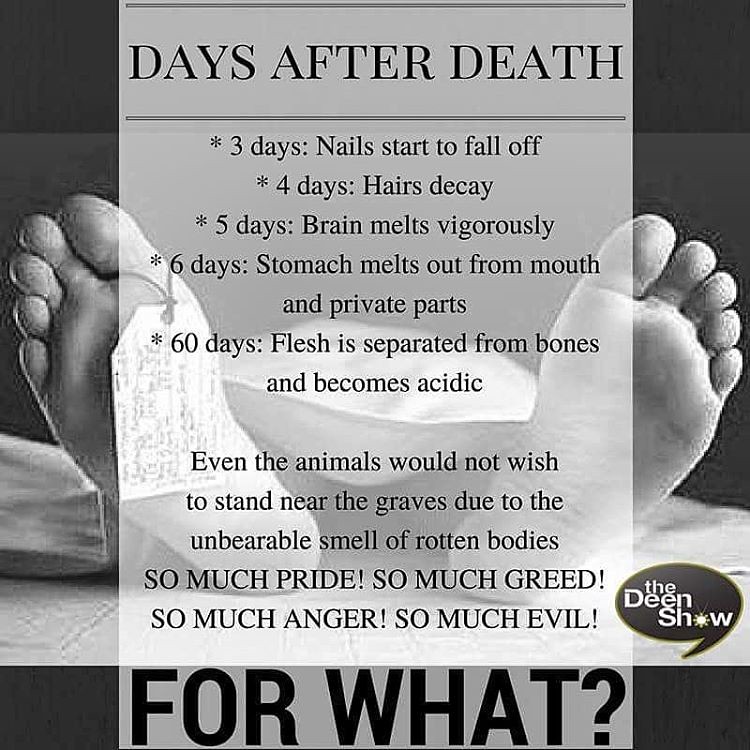This horizontally aligned poster features a striking grayscale image of two bare feet, viewed from the soles, peeking out from under a white sheet, lying on a bed. Superimposed upon this stark scene is a semi-transparent gray square with a black banner at the top. In uppercase Times New Roman font, prominently at the top it reads "DAYS AFTER DEATH." Below this title, against a black horizontal line, the poster lists in progressively smaller but centered text: 

- *Three days: nails start to fall off.*
- *Four days: hair decays.*
- *Five days: brain melts vigorously.*
- *Six days: stomach melts out from mouth and private parts.*
- *Sixty days: flesh is separated from bones and becomes acidic.*

The text continues to detail the extreme decomposition process, noting: "Even the animals would not wish to stand near the graves due to the unbearable smell of rotten bodies."

Following this grim enumeration, the poster dramatically states in expanding uppercase letters, "SO MUCH PRIDE! SO MUCH GREED! SO MUCH ANGER! SO MUCH EVIL!" centered on separate lines.

A black banner at the bottom transforms into gray and dominantly asks the question "FOR WHAT?" in the largest uppercase text. Near the lower right corner, a black quote box with white text credits "The Deen Show."

The image and accompanying text seemingly aim to deliver a poignant message on mortality and the futility of egotistic pursuits, typical of a public service announcement or moralistic campaign by The Deen Show.